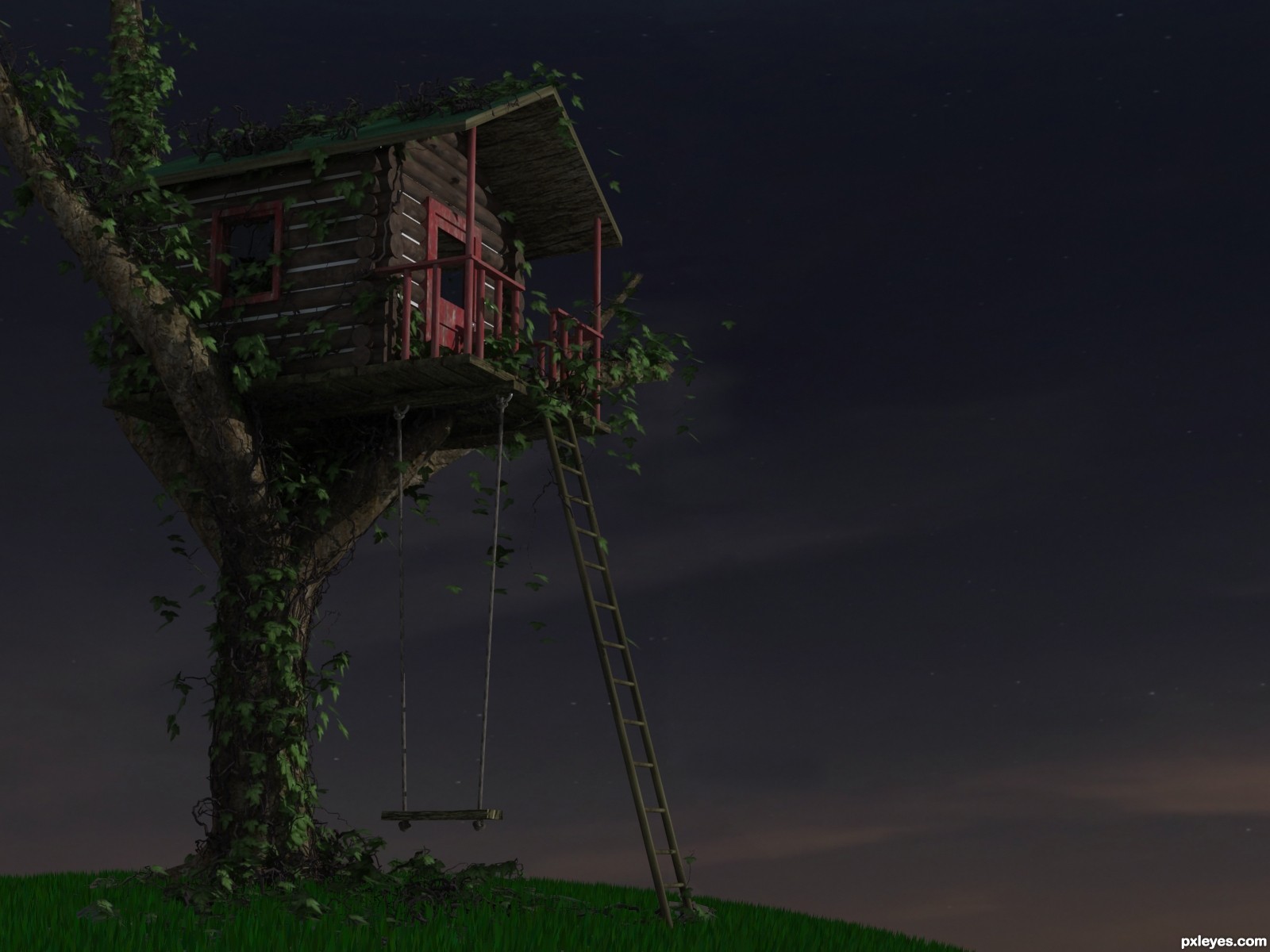This image, which appears to be a painting, depicts an atmospheric nighttime setting outdoors. The scene is rendered in such dark tones that visibility is limited, with the background almost completely black. Centrally featured is a small tree house perched within the branches of a Y-shaped tree covered in ivy. The tree house, built from logs, showcases a red door with a square window and a porch with red railings. The porch sits high above the ground, accessible by a long ladder that stretches diagonally downward. Additionally, a rope swing with a wooden seat hangs from the underside of the tree house. In the lower right corner, small white text reads "p-x-l-e-y-e-s dot com." The composition includes subtle elements such as brown-tinted clouds blending into the night sky and patches of green grass, suggesting the setting is atop a hill. The top portion of the image remains enveloped in solid black, with a faint outline of additional trees possibly visible. White light shines faintly through the wooden planks of the tree house, enhancing its almost ghostly silhouette against the dark backdrop.